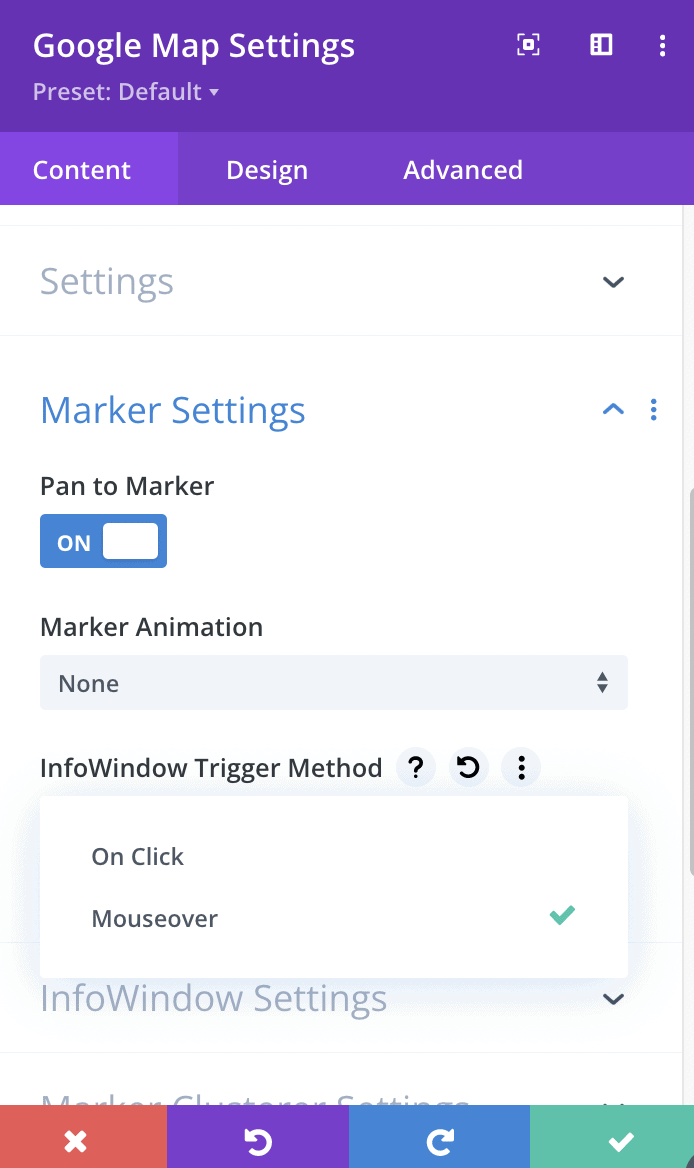The image shows the Google Maps Settings page featuring a prominent bluish-purple banner at the top, labeled "Google Map Settings." Directly below this is a dropdown menu indicating "Preset Default." 

Beneath the banner are three side-by-side tabs: "Content," which is highlighted in a slightly lighter color, "Design," and "Advanced." Below these tabs, the page is organized into multiple sections.

The first section reads "Settings" with an accompanying dropdown arrow. Below this is another section titled "Marker Settings," displayed with an upward-pointing arrow next to it. Under "Marker Settings," the text "Pan to Marker" is shown alongside a blue rectangular button labeled "On."

Following this, there is "Marker Animation," accompanied by a text box containing the word "None." Next, the page reads "Info Window Trigger Method," which includes a question mark, a circular-arrow icon, and three vertical dots. Below this, "On Click" is displayed, with "Mouse Over" and a check mark beneath it.

Lastly, the "Info Window Setting" section is located, and at the bottom of the page are four colored rectangles: a red rectangle with a white "X," a purple rectangle with a left-pointing circular arrow, a blue rectangle with a right-pointing circular arrow, and a green rectangle featuring a white check mark.